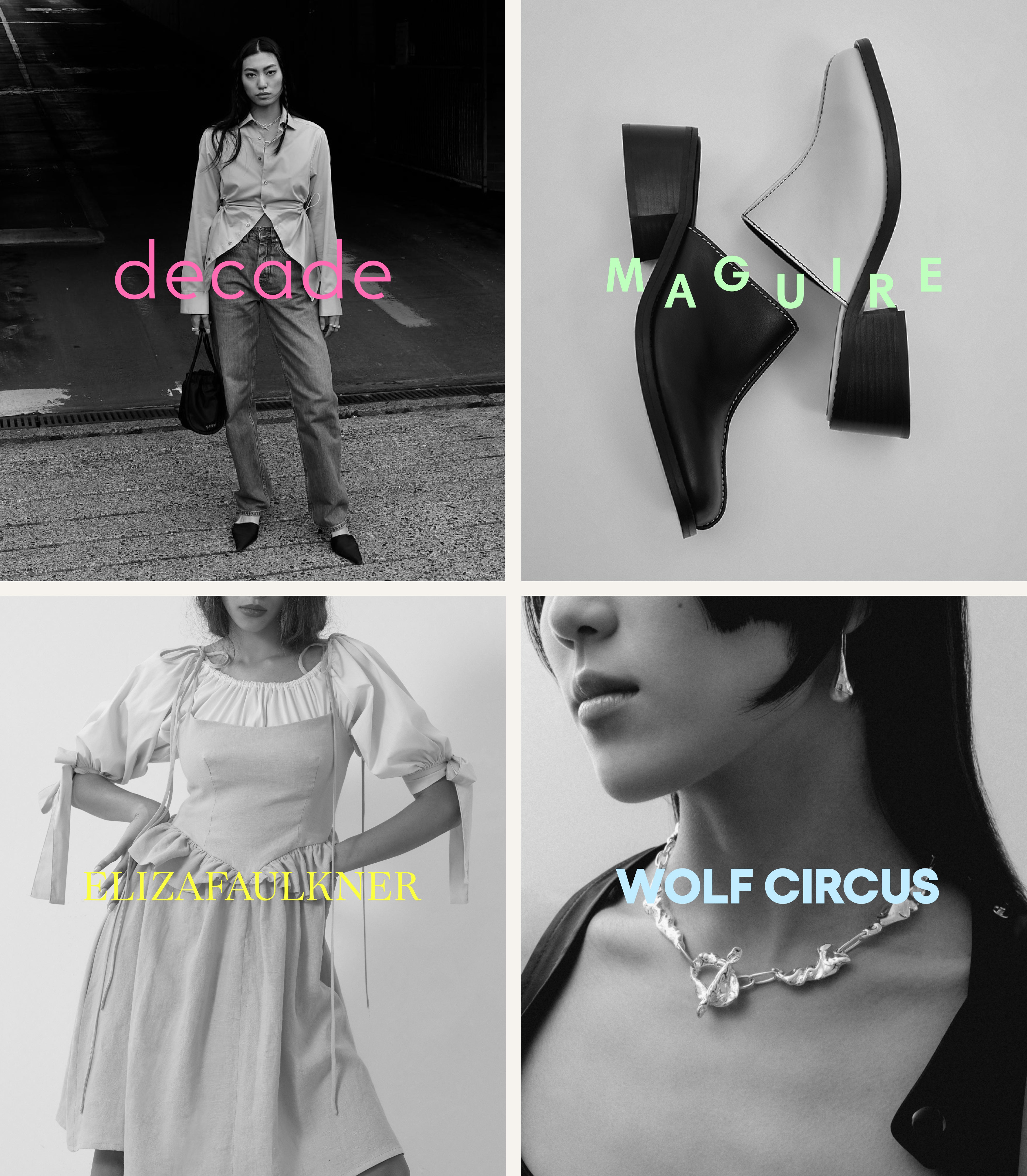The image is a composite of four black and white photographs arranged in a large square with a white border separating each section. 

- **Upper Left:** A woman in a business-casual outfit, consisting of trousers and a button-down shirt, carries a black bag and wears pointed shoes. The word "DECADE" is written in pink letters across her waist.
- **Upper Right:** A pair of slip-on shoes, one black and one white, both featuring thick black heels, placed on a light gray surface. The text "MAGUIRE" accompanies this image.
- **Lower Left:** A woman dressed in a jumper with a white shirt adorned with long bows at the elbows. The name "ELIZA FAULKNER" appears twice in yellow, all-caps text across the center of the image.
- **Lower Right:** An image focuses on the lower part of a woman's face, neck, and chest, showcasing a large silver necklace and a drop earring. "WOLF CIRCUS" is written in light blue letters across the center.

Overall, the detailed descriptions merge to showcase each photograph's distinctive elements and accompanying brand names, emphasizing their advertisement nature.